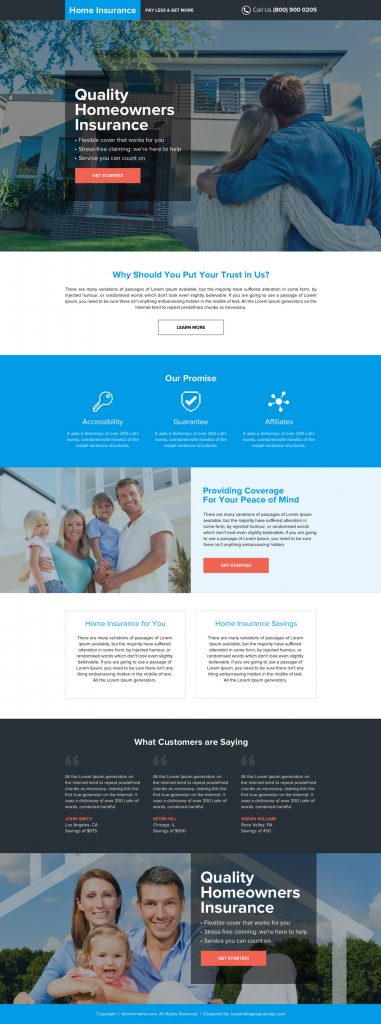The website features a black or dark gray header prominently displaying "Home Insurance" in blue text on the left side. Adjacent to this, to the right, there is additional small white text that is difficult to read. A "Call Us" button with a phone icon inside a circle is also present, followed by a phone number in bold white font.

Below the header, the main image showcases a man in a blue collared shirt with his left arm around a woman with blonde hair wearing a white sweater. They are gazing up at a windowed area of a white, square-shaped house. 

In the foreground, a transparent black notification panel appears with the bold white text "Quality Homeowners Insurance." Below this notification, three bullet points highlight the benefits of the insurance. Next to these, there is an orange rectangular icon with white text.

Further down the page, a section with a white background poses the question "Why should you put your trust in us?" in bold blue lettering, followed by explanatory text in smaller black font. This section includes a white rectangle bordered in black that features "Learn More" in bold black capital letters.

At the bottom, a blue background banner displays three white icons: a key on the left, a shield with a check mark in the center, and a network icon on the right, with the label "Affiliates" underneath.